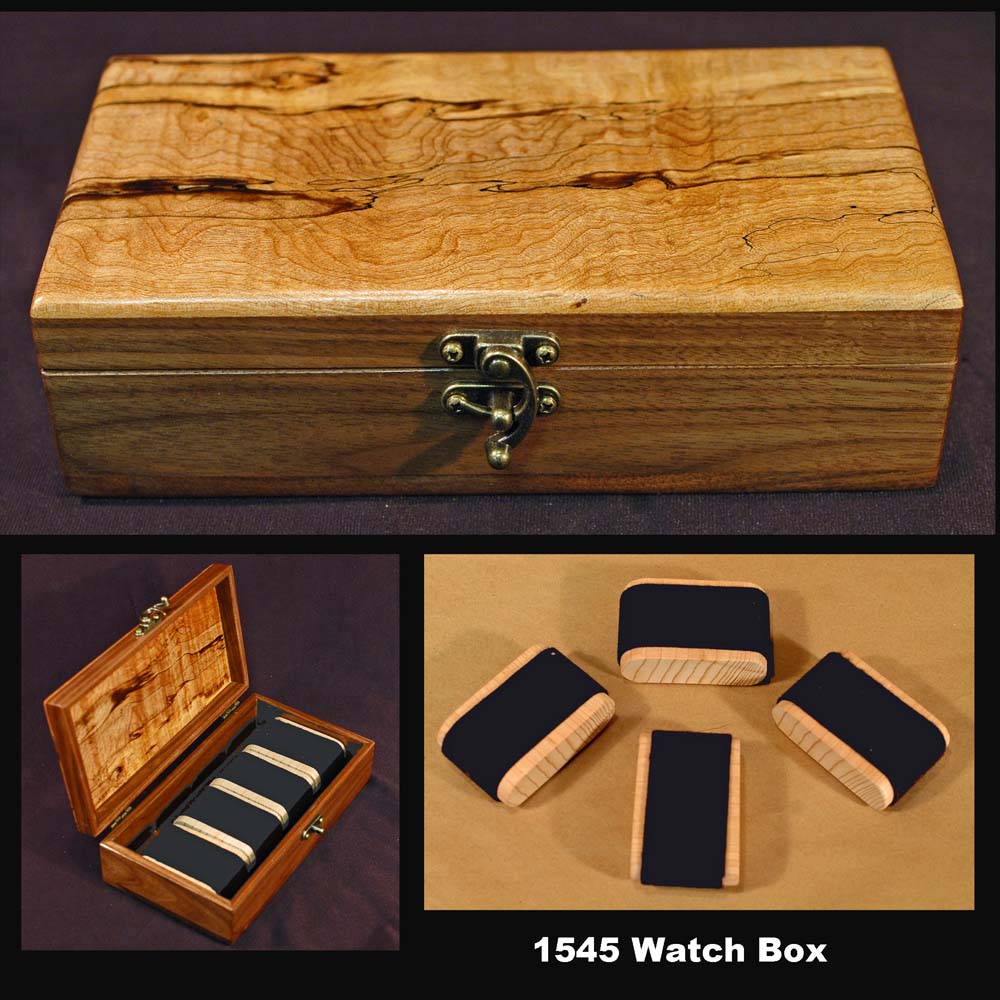This professional product image features the 1545 Watch Box and is set against a dusky maroon backdrop. At the top of the image, the closed watch box is displayed. Crafted from light natural wood with subtle reddish-brown patterning and a metal clasp closure, the box rests on a rich maroon felt surface. Below this, the box is shown open, revealing its wooden interior lined with four removable black felt-covered blocks designed to securely hold watches. The wood inside matches the outer wood, and additional details highlight the meticulous construction. Finally, a close-up shot displays the four cedar wood blocks, each wrapped in black felt, arranged in a neat formation. In white lettering below these images, the text reads "1545 Watch Box."